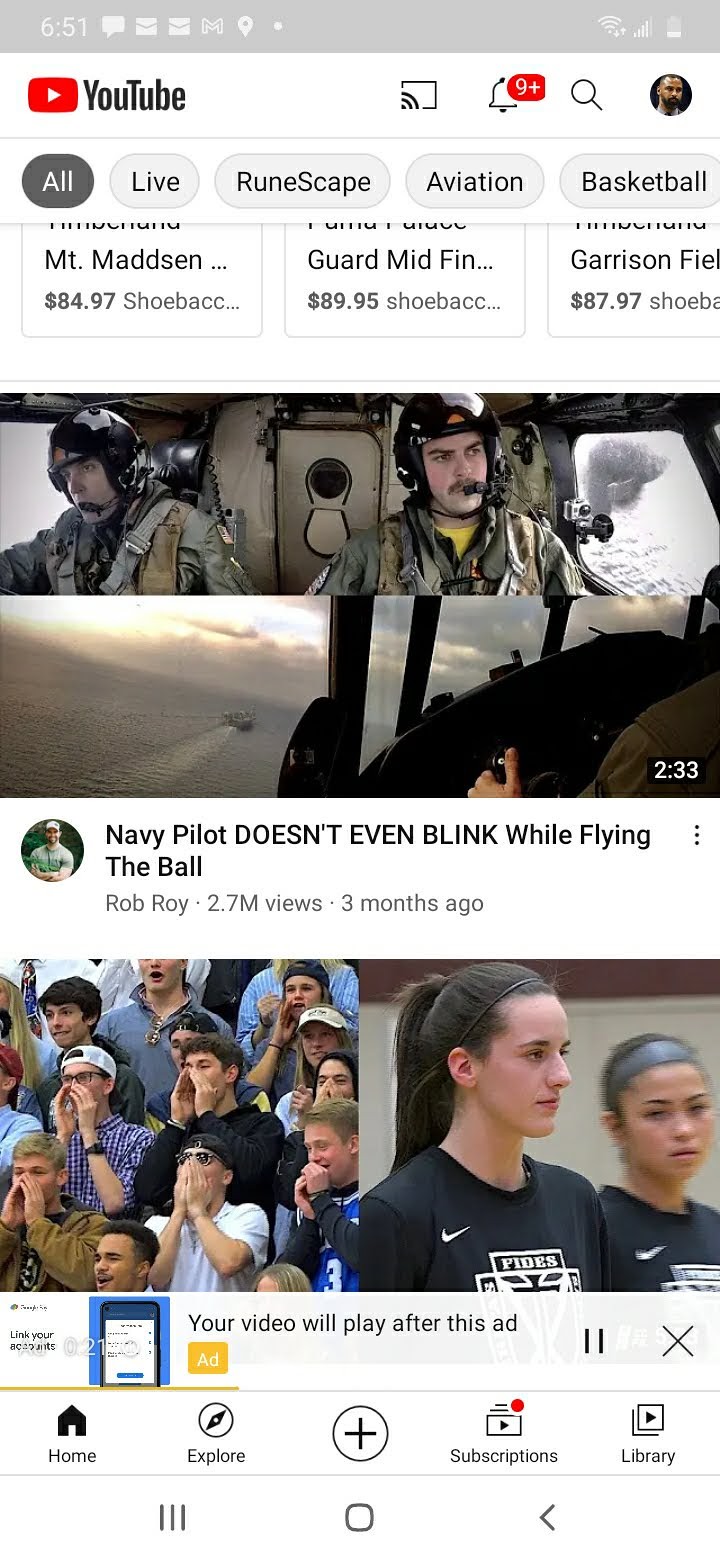The image depicts a YouTube mobile home page, characterized by its tall rectangular shape with smartphone interface elements like the Wi-Fi symbol, messaging symbols, and the time at the top. The YouTube logo, consisting of a red rectangle with a white triangle and the bold black text "YouTube," is prominently displayed on the upper left. 

The primary content highlighted in the feed includes two main videos. The top video, titled "Navy Pilot Doesn't Even Blink While Flying the Ball," posted by Rob Roy three months ago, boasting 2.7 million views, features a split image: the upper section shows two aviators wearing helmets and military fatigues, while the lower section captures a dramatic scene of a jet aircraft approaching an aircraft carrier at dusk. 

Below this video is another entry featuring two athletes, likely Caitlin Clark and a teammate, both in black Nike uniforms with distinctive logos. Adjacent to them is a vibrant crowd scene, with several men energetically calling out, some cupping their hands around their mouths to amplify their voices. The bottom interface of the YouTube home page includes navigation options like the home, explore, subscriptions, and library buttons.